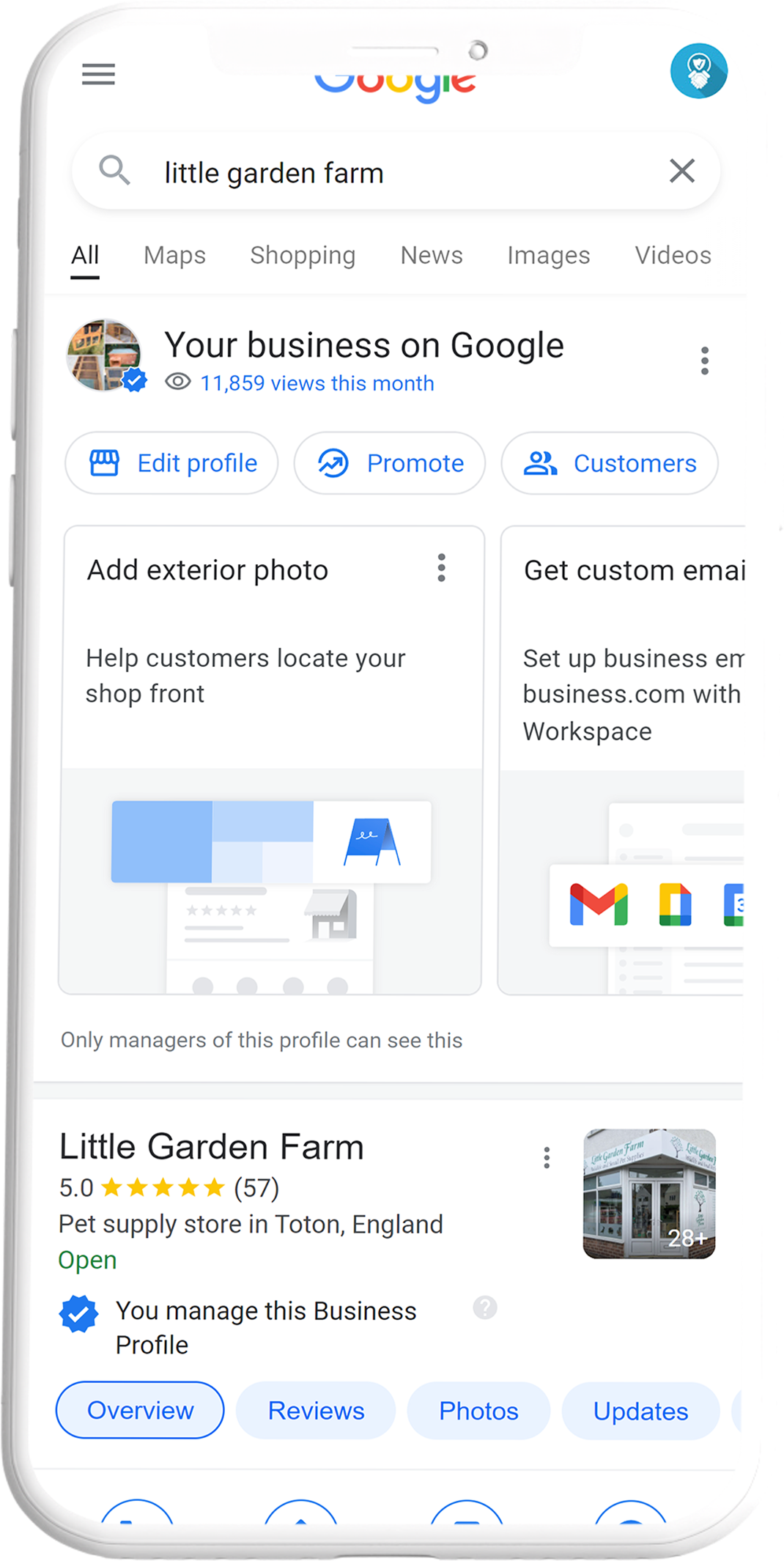The image displays a Google My Business profile page for "Little Garden Farm," set against a white background. At the top, three black lines serve as a menu icon. The word "Google" appears prominently in blue, red, yellow, and green colors. Below this, there is a blue circle containing a person icon, followed by a search box with the text "Little Garden Farm."

Navigation options—All, Maps, Shopping, News, Images, and Videos—are displayed beneath the search box, with "All" underlined to indicate it is selected. 

Further down, a section labeled "Your Business on Google" includes a blue circle with a check mark, noting "11,859 views this month." Adjacent to this are three dots indicating more options.

The interface continues with three blue buttons: "Edit Profile," "Promote," and "Customers." Below this, a large box invites the user to "Add Exterior Photo" with a suggestion to "Help Customers Locate Your Shop Front," accompanied by three dots for extra options. It also informs that "Only Managers of This Profile Can See This."

To the right, a box labeled "Get Custom Emails" promotes business email setup with Google Workspace, including an illustrative image.

The next section features a detailed profile of "Little Garden Farm," identified as a pet supply store in Toton, England, with a five-star rating. The business status is marked as "Open," and it includes an affirmation that "You Manage This Business Profile" with a blue check circle and more options via three dots. A picture of the business' front is shown, paired with a small light blue circle containing a question mark for additional help.

At the bottom, four blue buttons labeled "Overview," "Reviews," "Photos," and "Update" link to different sections of the profile. The layout concludes with the visual of four partially visible semi-circles cut off at the bottom of the screen.